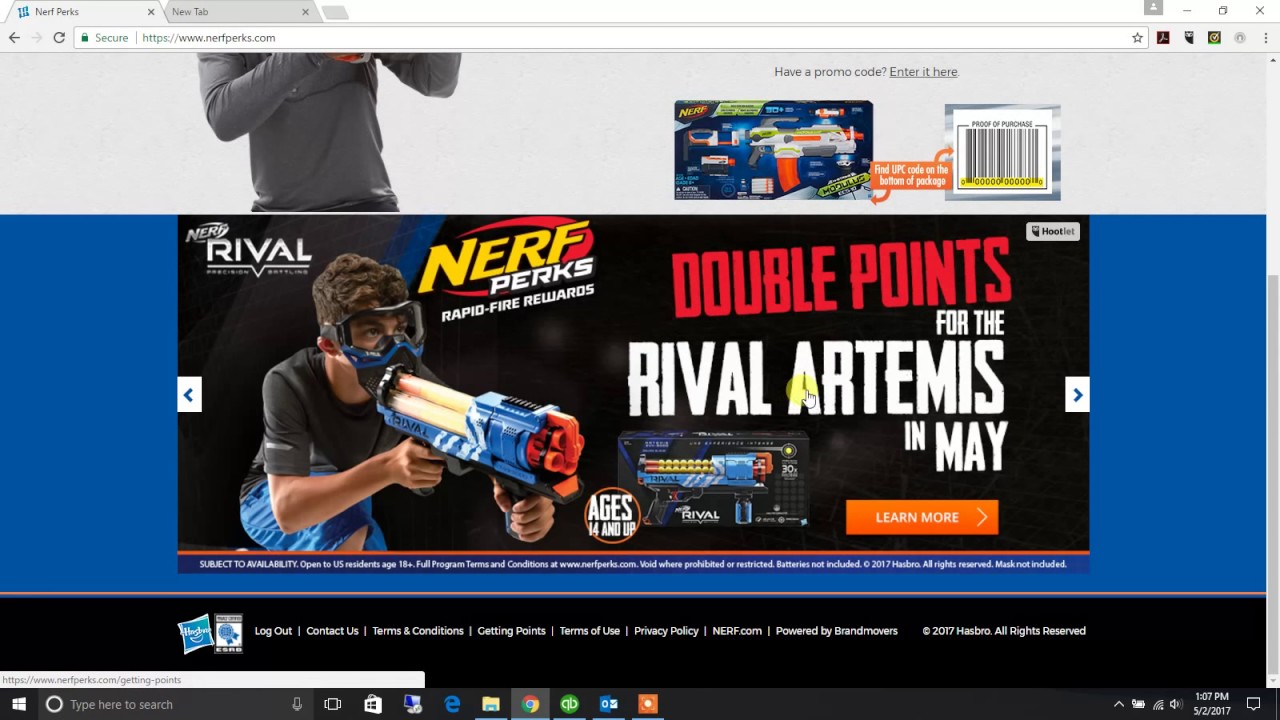Screenshot of a promotional webpage featuring a special offer for Nerf products. The banner headline at the top of the promotion reads "Nerf Perks: Rapid-Fire Rewards." Below this, there is an image of a young boy holding a large Nerf rifle. To the right of the boy, bold text announces "Double Points for the Rifle Artemis in May." Below this information is a vibrant orange box with the text "Learn More" inviting users to explore further details. The URL and the titles of two open browser tabs are visible at the top of the window, though they are too small to be clearly discerned.